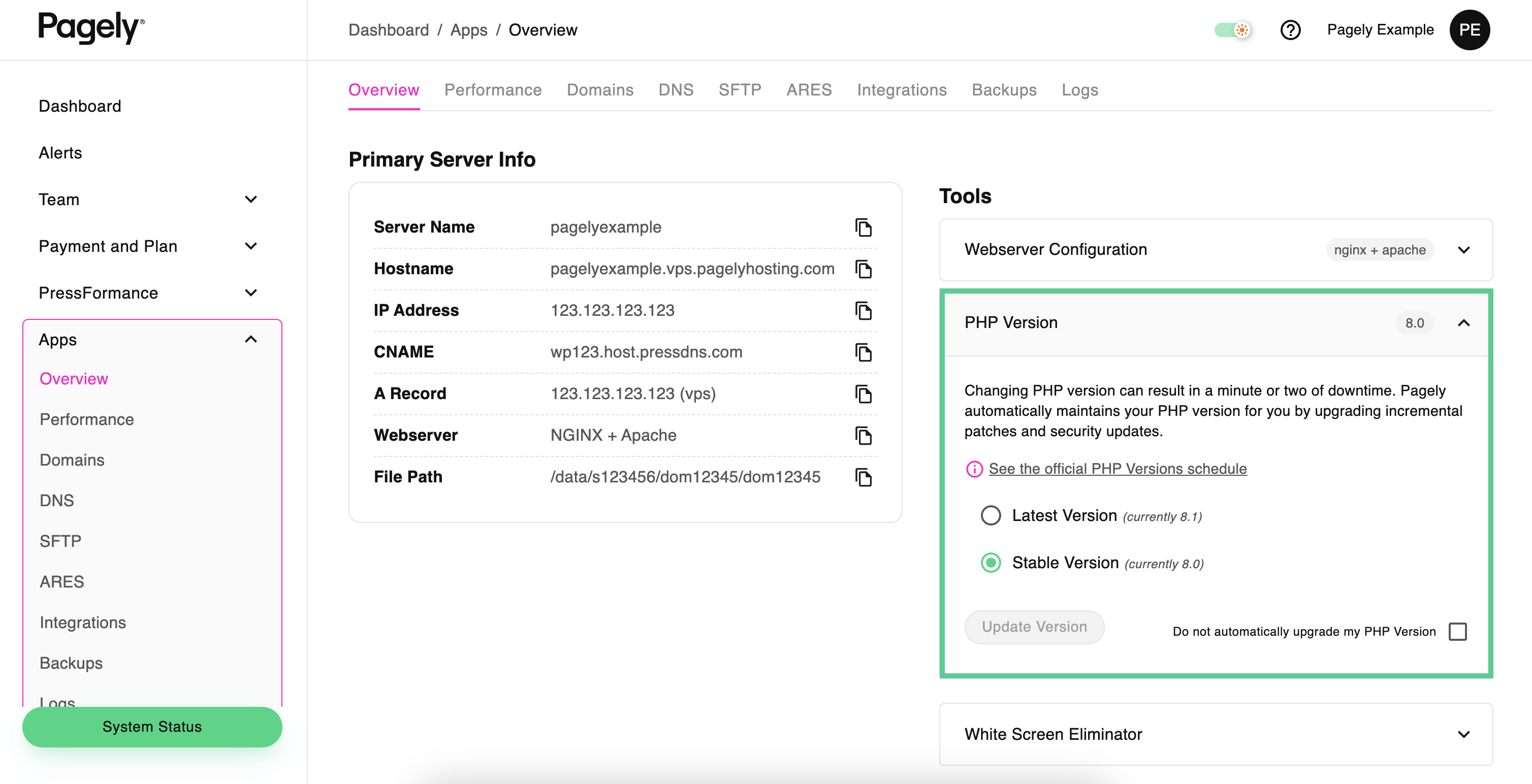The image displays the Pagely Dashboard's Apps Overview section. On the left side of the interface, there's a vertical navigation menu listing various sections in descending order: Dashboard, Alerts, Team, Payment and Plan, Press Performance, Apps, Overview, Performance, Domains, DNS, SFTP, ARES, Integrations, Backups, and at the very bottom, a green button labeled "System Status."

In the central area of the dashboard, there's a horizontal menu bar at the top with tabs for Overview, Performance, Domains, DNS, SFTP, ARES, Integrations, Backups, and Logs. Below this menu, detailed information about a primary service is displayed. This includes:

- Server IMSO
- Server Name: Pagely Examples
- Host Name: Pagely Example at vps.pagelyhost.com
- IP Address: 123.123.123.123
- CNAME: wp123.host.pressdns.com
- A Record: 123.123.123.123.vps
- Web Server: NGINX plus Apache
- File Path.